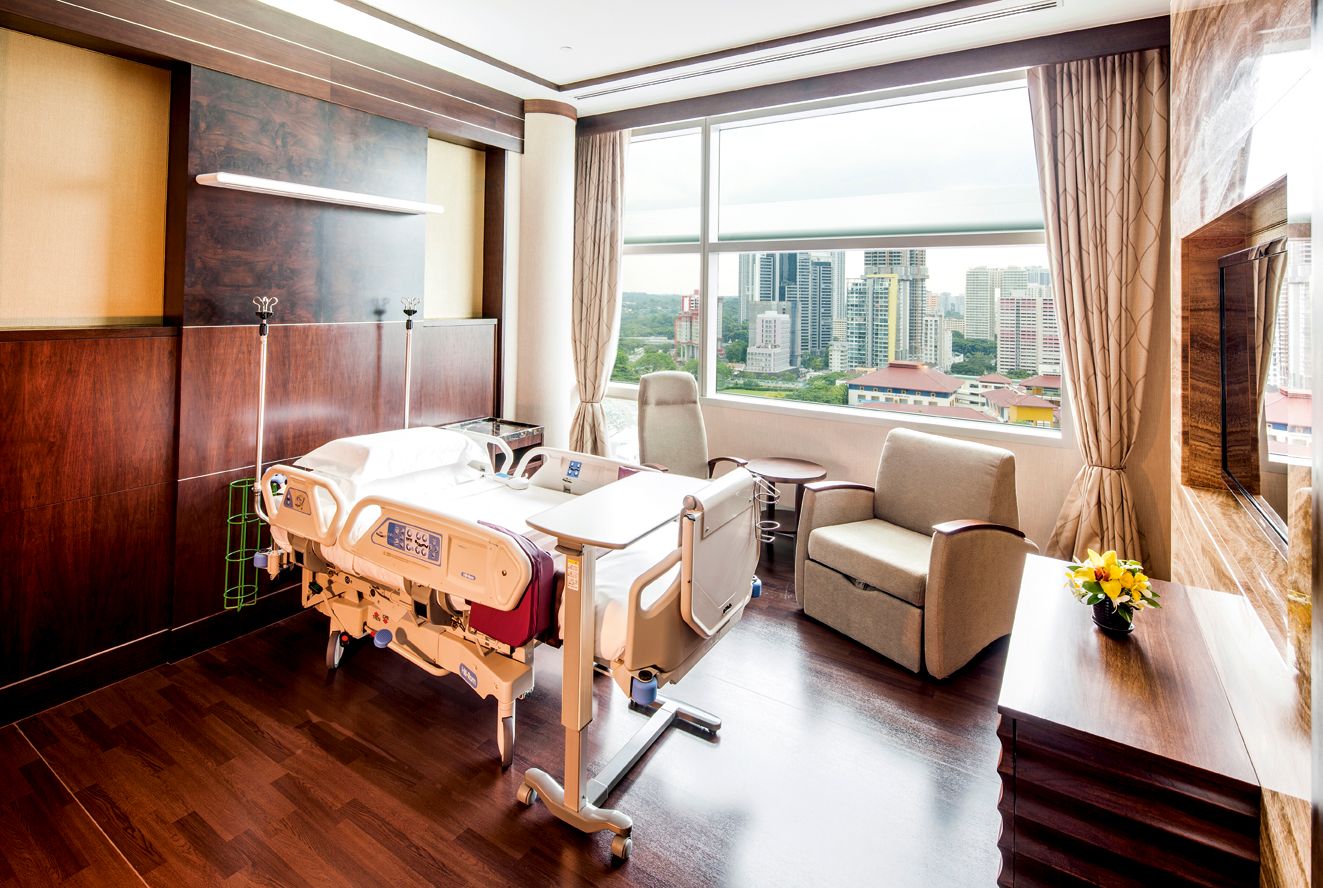The image captures an elegantly designed room that appears to serve as a high-end hospital room, merging healthcare functionality with the comforts of a luxurious living space. At the center of the room is a hospital bed equipped with adjustable features and a movable tray, indicating its medical purpose. The room is warmly decorated with rich wooden floors and paneling, contributing to its homely ambiance. A large picture window towards the back offers a pretty outdoor view, flanked by two comfortable sofas that provide seating for visitors. There's a television attached to the wall on the right side, adding to the room's modern amenities. Below the television, a small drawer is topped with flower pots sporting yellow and green petals. The decor is marked by a palette of brown, beige, white, red, green, and various shades of yellow and green. The overall setting is devoid of any textual elements, underscoring the room’s peaceful and inviting atmosphere.